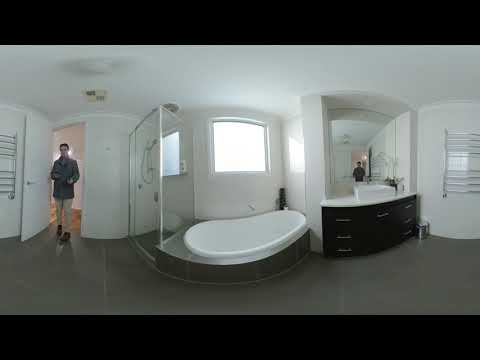This panoramic image portrays a sleek, modern bathroom with a clean, minimalist design. Starting from the left, a person wearing khaki pants and a gray coat stands just inside an open doorway, holding a pole, likely for taking the picture. Adjacent to this person is a clear glass shower stall, providing a clear view inside and featuring a window within the shower space. Beside the shower is a large white bathtub, which sits sunken into a floor of concrete gray tiles that match the rest of the bathroom floor. Above the bathtub, there is a prominent window, adding a sense of openness to the space.

On the right side of the bathtub, a dark-colored vanity with several drawers and silver handles houses a raised square sink. This vanity is crowned by a large mirror, which reflects another indistinct figure in the bathroom. The right-hand side wall is adorned with a vertically stacked array of silver towel racks.

The bathroom’s walls are a crisp white, contrasting neatly with the dark gray floor, and the ceiling is also white, contributing to the room's bright and airy atmosphere. Overall, the room exhibits a sophisticated aesthetic with its combination of white and dark gray elements, clear glass, and reflective surfaces.